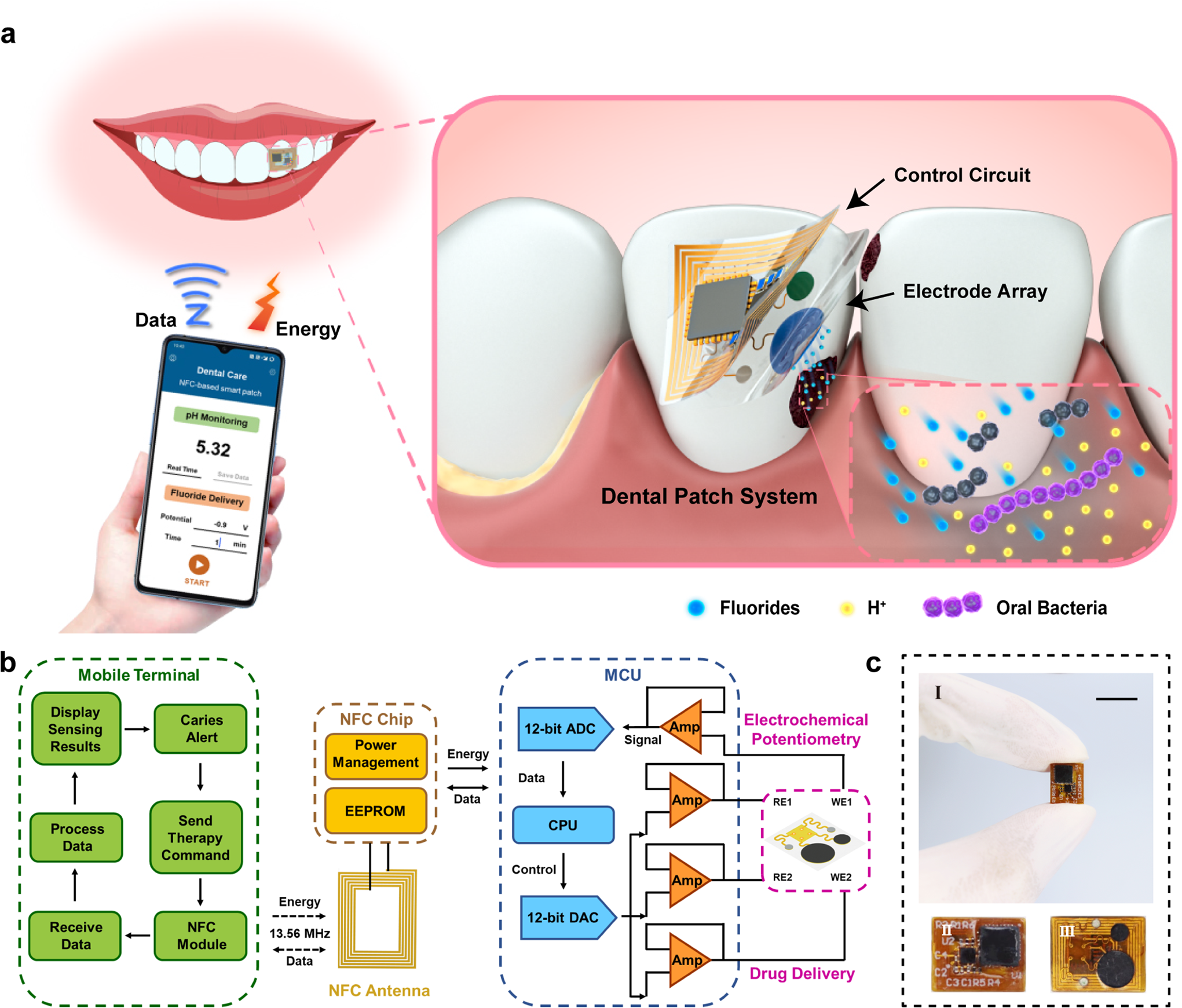The infographic illustrates a sophisticated dental patch system designed to deliver fluoride and monitor oral health. On the left side, labeled "A," there's a diagram featuring a woman's mouth with red lips and white teeth, highlighting a small patch on an incisor tooth. Below the mouth, a smartphone app display is depicted, syncing with the dental patch system. The app monitors various parameters, including fluoride delivery and energy transmission, indicated by blue radio waves and a red lightning bolt. The app interface shows a figure of 5.32 and a start button, although some details are too small to read.

Adjacent to this, there's an enlarged view of the dental patch, showcasing the control circuit and electrode array. The patch appears as a tiny computer chip, likely affixed to the tooth's surface. Underneath, in Figure "B," a flow chart details the process from sensing results on the mobile terminal to caries alert and SAN therapy command, involving an NFC module for data exchange. The energy required, set at 13.56 megahertz, facilitates communication between the NFC chip and the MCU flow chart, which integrates 12-bit ADC and DAC for signal processing.

Further elements include an electrochemical potentiometry system, registering data for drug delivery. The lower section, marked "C," portrays a human hand holding the diminutive chip, roughly the size of a fingernail, and provides an enlarged view of both its front and back sides. The infographic uses color codes in blue, yellow, and purple to demarcate various stages of the process and technical elements, providing a comprehensive visual representation of the dental patch system's functionality.